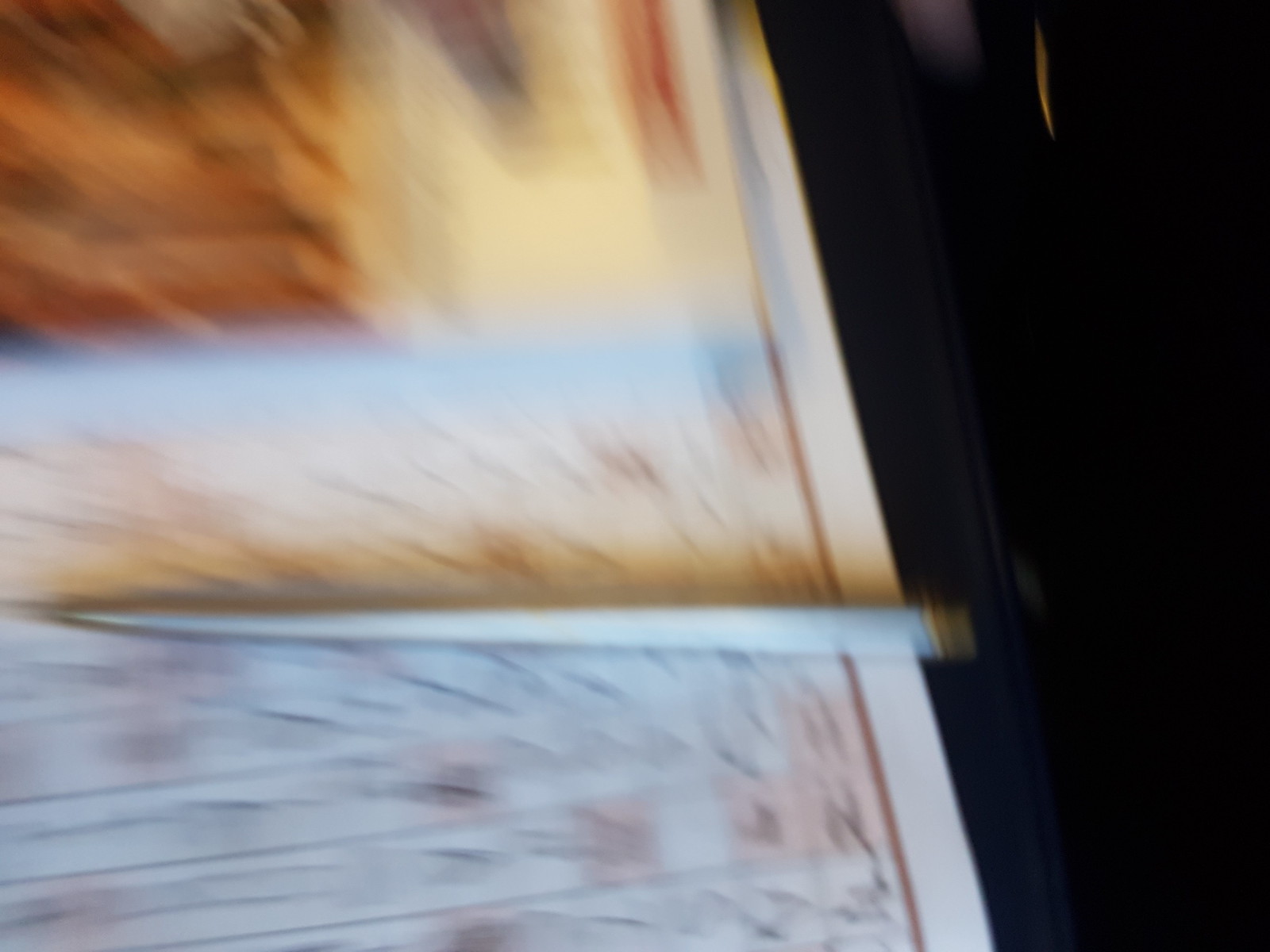A horizontal, heavily blurred image captures a vertical object divided into multiple sections distinguished by various colors. The object is framed with a brown border, which is further outlined by a thin white border. Within the main object, a pencil-like figure is positioned diagonally, with its pointed end near the center-left and extending approximately three-quarters of the way to the center-right. Due to the intense blurriness, the specific contents within the colored sections, boxes, and rows are indiscernible. The entire composition rests against a uniformly black background.